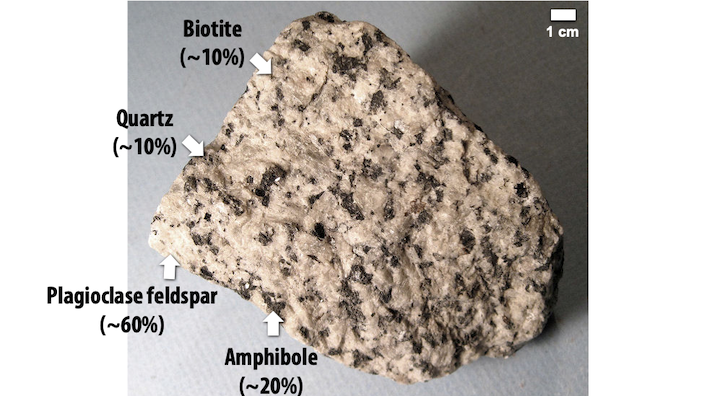The image depicts a close-up of an irregularly shaped rock with a predominantly gray color interspersed with black specks of varying sizes. The rock is positioned on a light, textured surface, with the lighting source coming from the lower left, which creates a shadow in the upper right, resulting in a lighter lower right and dark gray upper right background. The rock itself is flat at the left and bottom edges, while the right side and top edge are jagged and curved, almost reaching the top of the image before curving down and to the left.

Four white arrows label different mineral components of the rock: "biotite (10%)" at the top left, "quartz (10%)" below on the left, "plagioclase feldspar (60%)" on the bottom left in a very light area, and "amphibole (20%)" on the bottom right in a darker spot. In the upper right corner, a small white rectangle serving as a scale indicates "1 cm."

This detailed image provides a clear and well-lit view, highlighting the rock's composition and surface texture.